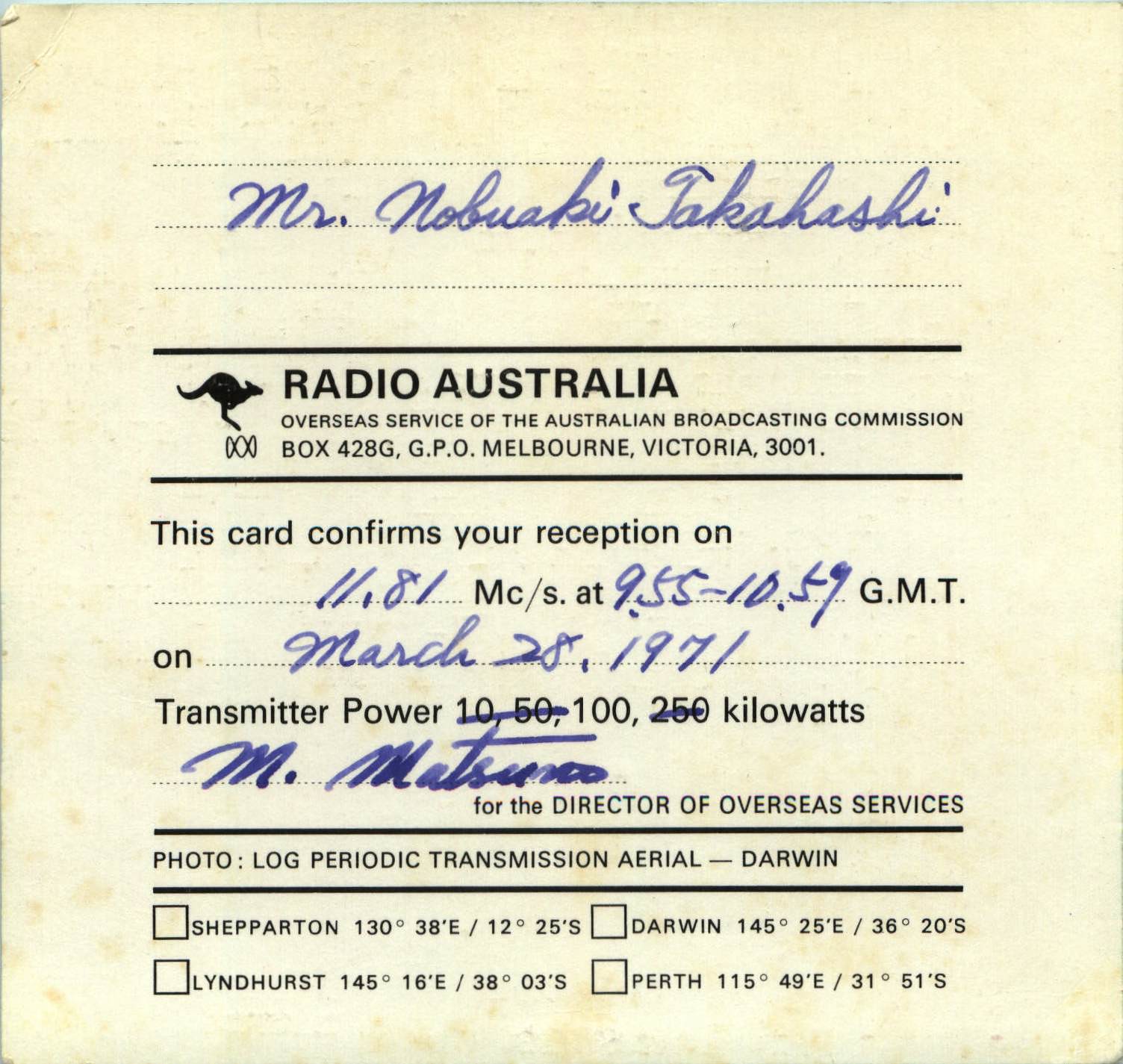This image features an aged reception confirmation card from Radio Australia, prominently displaying the text "Radio Australia" in bold black letters at its center. At the top, in handwritten blue pen, the recipient's name, "Mr. Nobuyuki Takahashi," is inscribed. The card details the confirmation of radio reception on the frequency 11.81 MCS at 955-1059 GMT on March 28, 1971, with a transmitter power of 100 kilowatts. The confirmation is signed by M. Matsumo on behalf of the Director of Overseas Services. Additional text in black indicates, "Photo, Log, Periodic Transmission, Aerial, Darwin," and includes coordinates listed for Sheperton, Darwin, Linhurst, and Perth. A logo for Radio Australia featuring a kangaroo silhouette, along with the address for the Australian Broadcasting Commission, is also present, giving the document an official appearance reminiscent of dated internal documentation.